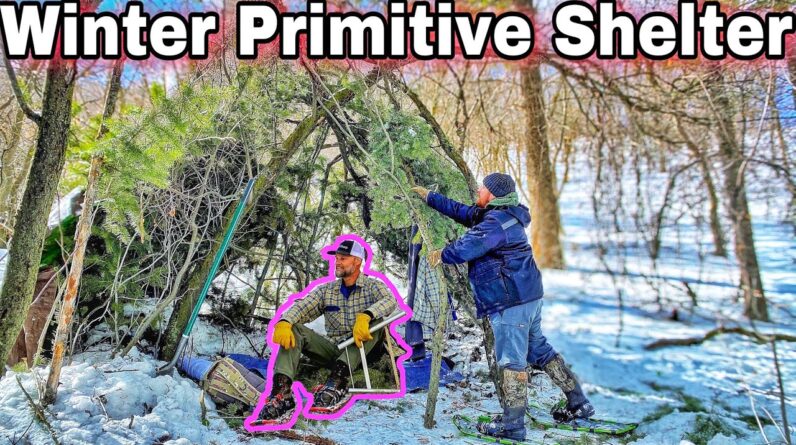Under the title "Winter Primitive Shelter" in large white block letters with black outlining, the photo captures a winter scene deep in a snowy forest filled with dead trees and evergreen branches. Two men are working together to construct a makeshift tent from tree limbs. The man standing is dressed in an all-blue ensemble, including a blue jacket, blue jeans, and a blue stocking hat, with knee-high camouflage and black boots. He is seen gathering loose branches from the surrounding trees. 

The second man, outlined in a magenta-pinkish-purple border as though sketched, sits on the snowy ground on a blue blanket. He is holding a white rod in his left hand and seems to be wearing green pants, black shoes, and a grayish plaid shirt. He also sports yellow gloves, a black baseball cap with a white back, and a smiling face directed to the left. Debris and dead wood litter the ground around them, while patches of blue sky peek through the forest canopy, suggesting a cold yet clear day. This detailed moment captures the early stages of their endeavor to construct a primitive winter shelter, with both men appearing focused and engaged in their task.